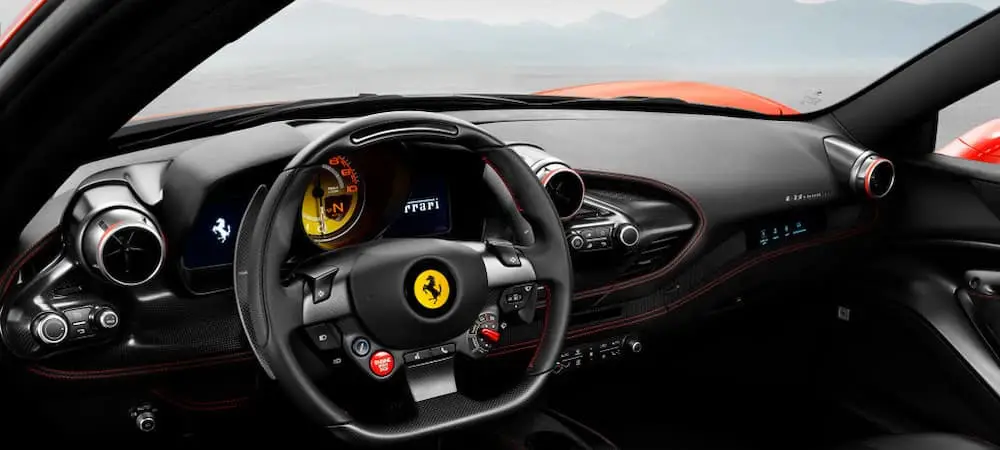This interior photograph of a Ferrari captures the sleek and modern design of the car’s cabin. The black interior is accented with red detailing, including red piping and borders on the premium leather surfaces. The steering wheel, which is flat at the bottom for ergonomic comfort, prominently features a bright yellow Ferrari logo with a rearing horse in its center, accompanied by a red engine start button. The dashboard is characterized by its smooth, aerodynamic contours and includes a yellow speedometer. The futuristic vents and digital elements enhance the modern feel of the space. From the driver's seat perspective, you can see the red exterior of the Ferrari through the curved windshield and partially see the side window, emphasizing the vehicle's striking color and design.